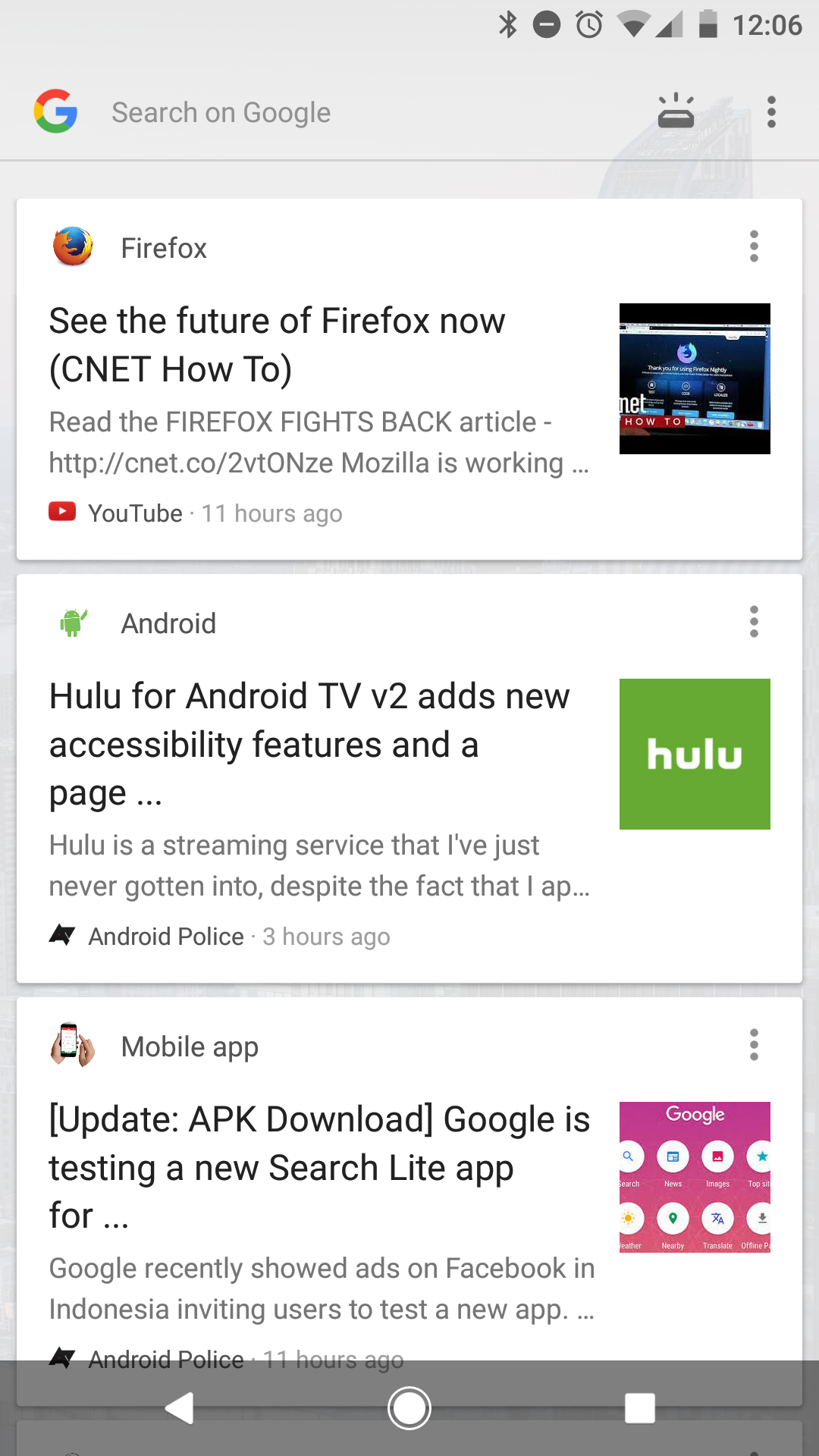Displayed on a smartphone screen is the result of a Google search. Various icons are visible at the top, including those for Bluetooth, an active alarm, Wi-Fi, and a signal strength indicator showing half bars. The battery icon indicates a 50% charge, and the current time is 12:06. Below these icons, there is a search bar labeled "Search on Google" accompanied by a three-dot dropdown menu.

The screen shows three distinct search results, each enclosed in a white rectangle. 

1. The first result features the Firefox icon and is titled "See the future of Firefox now (CNET How To)." Below it, there is a headline "Firefox fights back," followed by a YouTube link with the YouTube icon labeled "11 hours ago." The accompanying thumbnail image displays a computer screen primarily in black.

2. The second result focuses on Android and Hulu, titled "Hulu for Android TV v2 adds new accessibility features" from the source Android Police, published 3 hours ago. A green rectangle with the word "Hulu" in white is prominent in this section. This entry delves into new accessibility upgrades for Hulu's Android TV application.

3. The final result is about a mobile app update, titled "Update APK download: Google is testing a new search light app." It discusses Google's recent advertisements on Facebook in Indonesia, encouraging users to test a new application. The accompanying image features the Google logo set against a pink background, with eight small icons below it.

This detailed image not only showcases search results but also indicates various elements related to the smartphone's status and connectivity.